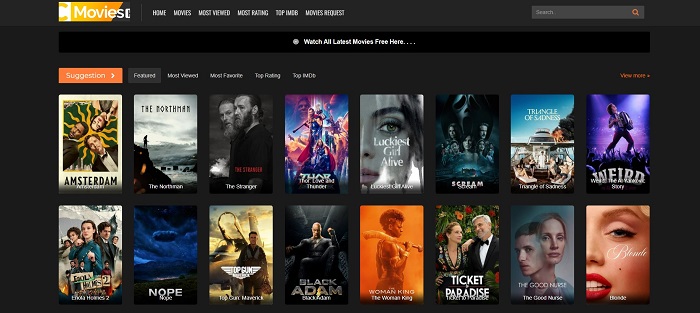This image is a screenshot of a website dedicated to movies. The website's theme is dominated by a sleek black background, which gives it a modern and cinematic feel. In the upper left corner, the name of the site, "Moviest," is prominently displayed. The name is written in a crisp white font over a slanted gold rectangle, adding a touch of elegance and style.

To the right of the site name, there is a navigation menu. While the fonts are somewhat small and a bit blurry, it’s evident that the menu items include "Home," "Movies," "Most Viewed," and "Highest Rating." There are two additional menu items, but their titles are unclear due to the image quality.

Centered at the top of the page, a bold statement reads, "Watch all the latest movies free here," enticing visitors with the promise of new content. Below this headline, there are two rows of movie posters, each row featuring approximately eight posters.

In the top left corner of the first row, the movie "Amsterdam" is prominently displayed. On the bottom row, towards the left side, the poster for "Ticket to Paradise," featuring George Clooney and Julia Roberts, is visible. Adjacent to it is the poster for "Woman King," followed by "Black Adam" and several other film posters. The consistent black background maintains the website's sophisticated aesthetic throughout.